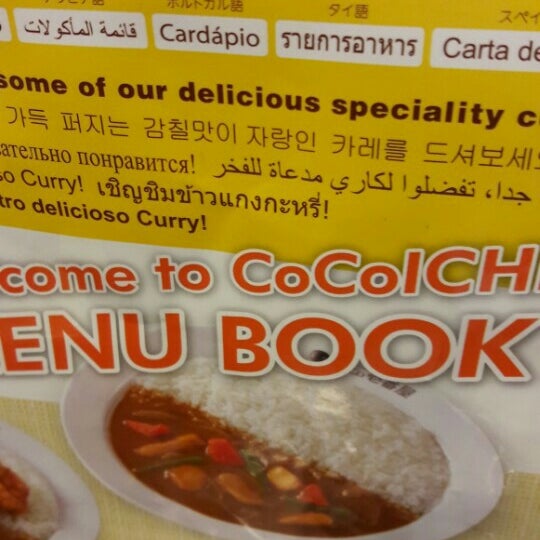The image is an extreme close-up of a restaurant menu from a curry place, featuring multiple languages. The background is a vibrant yellow with various translations of the phrase "some of our delicious specialty" prominently displayed in a brown font. The top section of the image has white rectangles with different categories written in various languages, including English, Arabic, Korean, and some Romance languages. Below this, the word "curry" appears twice, emphasizing the type of cuisine. There are also snippets of text in red, saying "Come to Cocoal CH," suggestive of the restaurant's name, potentially "Coco Ichiban," followed by "Menu Book." The bottom half showcases a dish: a white bowl with a perfectly divided presentation of white rice on the right and a vegetable stew or curry on the left, featuring a darker broth with baby carrots, potatoes, tomatoes, and possibly chicken. Another bowl is partially visible in the lower-left corner, hinting at more delectable offerings.